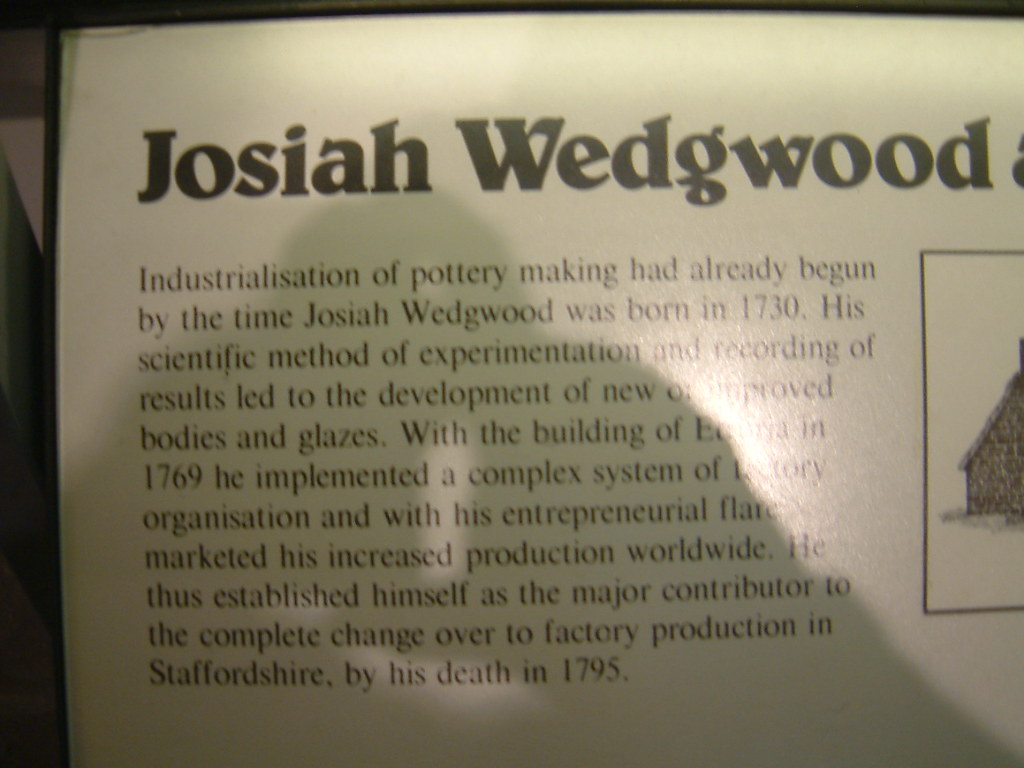The image appears to be a somewhat blurry photograph, possibly of a museum placard or newspaper clipping, featuring black text on a white background. The large heading at the top reads "Josiah Wedgwood." Below this, a block of text provides detailed information about Wedgwood's contributions to the pottery industry. Despite some glare obstructing parts of the text, key details are discernible. It explains that by the time Josiah Wedgwood was born in 1730, the industrialization of pottery making had already commenced. His use of scientific methods for experimentation and meticulous recording of results led to significant advancements in the development of new and improved pottery bodies and glazes. In 1769, with the establishment of an unspecified building (due to the glare), he implemented a sophisticated system of factory organization. His entrepreneurial skills facilitated the global marketing of his increased production. Wedgwood ultimately became a pivotal figure in the transition to factory production in Staffordshire, a legacy that was solidified by the time of his death in 1795. Additionally, the far right edge of the image shows a partial, possibly rectangular area with what seems to be a drawing of a house.